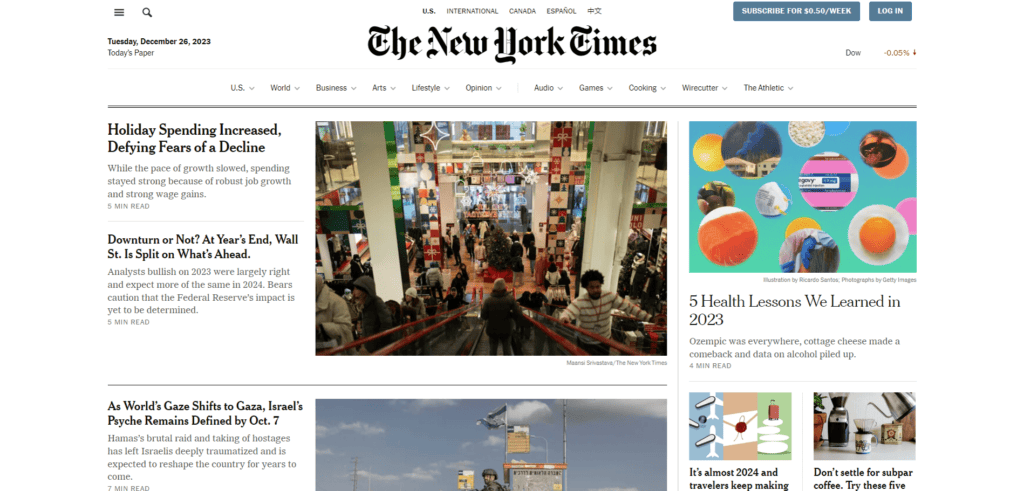The image is a horizontally rectangular screenshot of the New York Times website, captured on Tuesday, December 26, 2023. At the top-left corner, the date "Tuesday, December 26, 2023, Today's Paper" is visible. Centered at the top are navigation options labeled "U.S.", "International", "Canada", and "Español," providing users with diverse regional news selections. Directly below these options, the iconic New York Times heading stands out in its distinguished black font.

In the upper right corner of the website, there is a prominent "Subscribe for 50¢ per week" button next to a "Login" button, encouraging both subscriptions and account access. Directly beneath is a column on the left listing the day's headlines: "Holiday spending increased, defying fears of a decline," "Downturn or not, at year's end, Wall Street is split on what's ahead," and "As world's gaze shifts to Gaza, Israel's psyche remains defined by October 7th," showcasing the main stories.

At the center of the screenshot, two images are displayed. The left image captures the interior of a retail store, offering a bird’s-eye view from atop an escalator, possibly illustrating holiday shopping activity. To the right of these central images, additional visual content is presented, including a headline that reads "Five health lessons we learned in 2023," summarizing key health insights from the year. The comprehensive layout provides a snapshot of diverse news topics, designed to engage a wide readership.